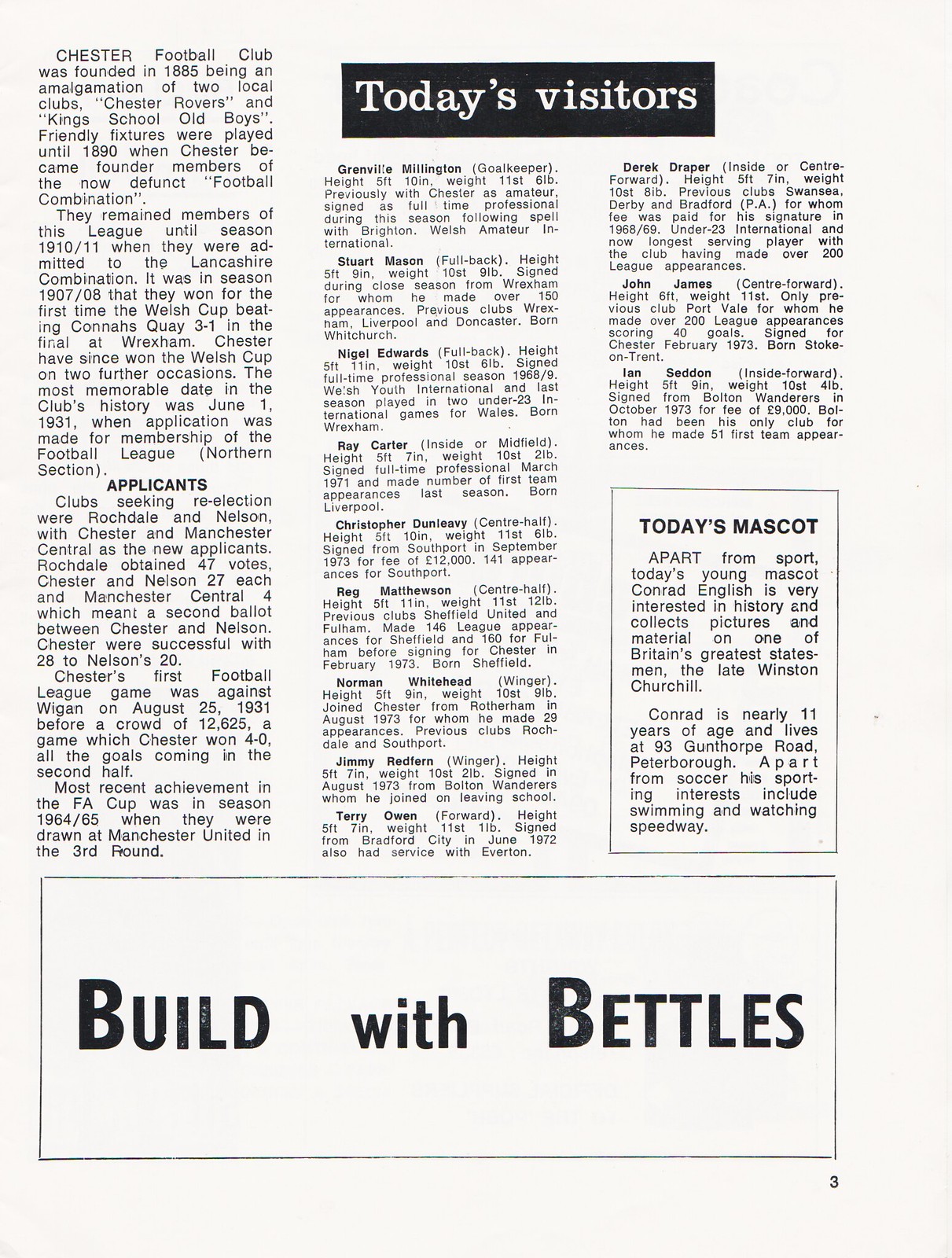This image appears to be a page from an older newspaper or gameday pamphlet. The background is white with black text. At the top of the page, a bold black banner reads "Today's Visitors." The page is primarily text, arranged in three columns. The left column begins with a detailed history of Chester Football Club, founded in 1885 as an amalgamation of Chester Rovers and King School Old Boys. It outlines the club's journey, including winning the Welsh Cup in the 1907-08 season and important milestones up to their first Football League game in 1931. 

The middle and right columns list names and soccer positions of the visiting team members, followed by a section on club applicants during a re-election period. Rochdale and Nelson were involved, with Chester ultimately securing enough votes to proceed. 

In the bottom right corner, there's a feature on today's mascot, Conrad English, a nearly 11-year-old boy who enjoys history and collects materials on Winston Churchill. Conrad also enjoys swimming and watching speedway. 

Spanning the bottom of the page is an advertisement in bold text that reads, "Build with Bettles."